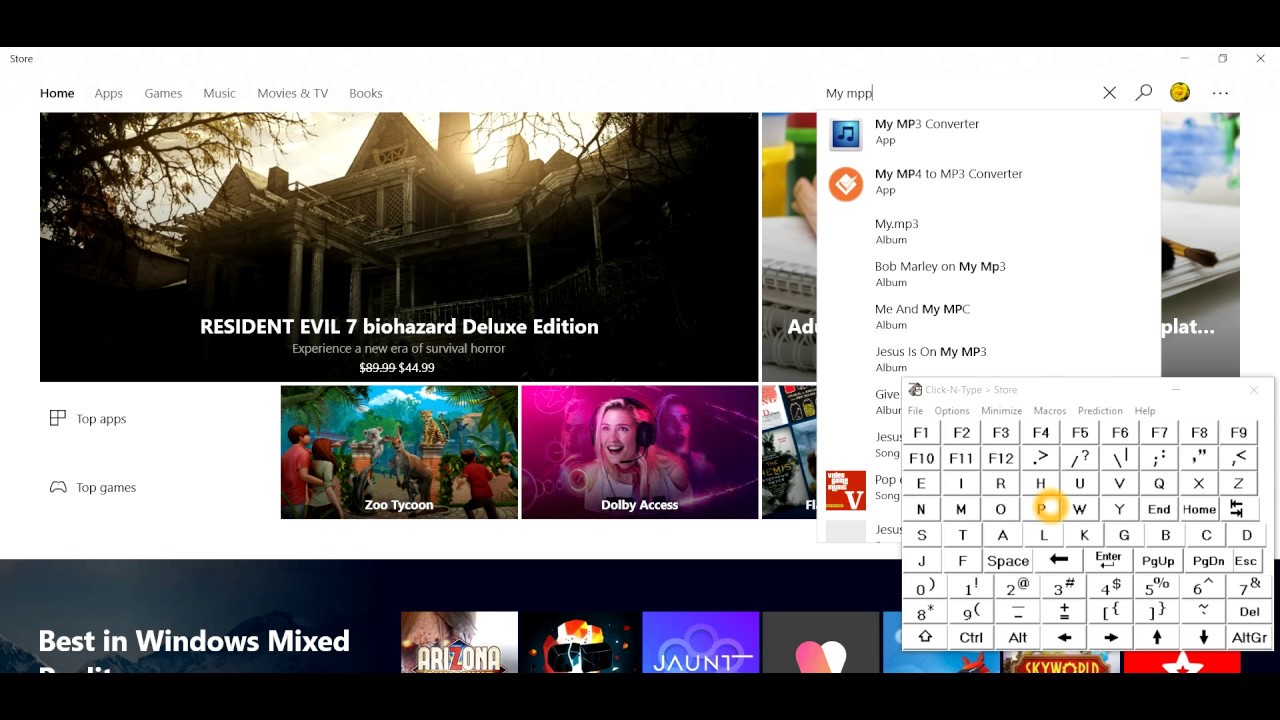This screenshot captures a view of the Windows Store on a web page, featuring black bars at both the top and bottom edges of the screen. The main content area boasts a white background. In the top left corner, "Store" is displayed in black font. Just below, there are navigation menus for Home, Apps, Games, Music, Movies & TV, and Books.

To the right of these menu options, there is an active search field where the user has typed "My MPP." This action triggers a dropdown menu suggesting a variety of available apps, including My MP3 Converter, My MP4 to MP3 Converter, My MP3 Album, Bob Marley on My MP3 Album, Me and My MPC Album, and Jesus on My MP3 Album.

Additionally, a peculiar white square on the screen features an open virtual keyboard that differs from the typical QWERTY layout, instead presenting the keys in alphabetical order. The letter "P" is distinctly highlighted with a yellow circle around it.